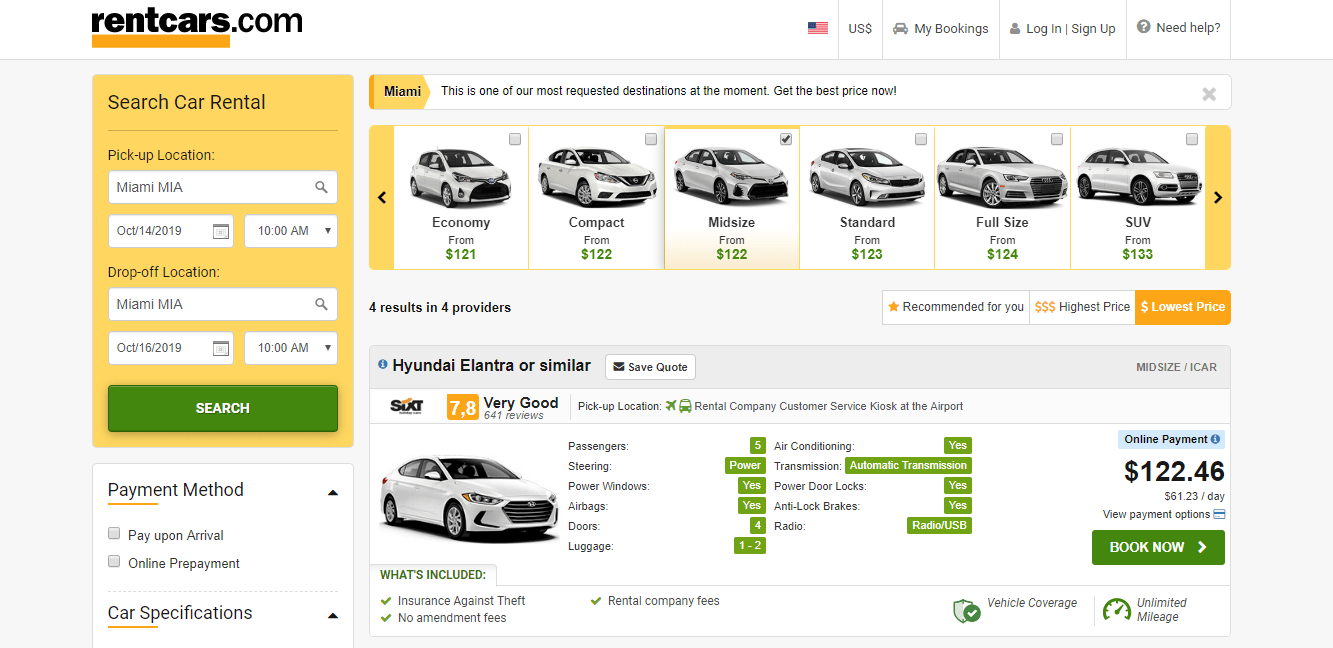In the image from rentcars.com, the logo "rentcars.com" is prominently displayed in bold, lowercase letters in the upper left-hand corner, underscored by a thick orange line. Towards the upper center-right, near the middle, there is an icon resembling the American flag followed by "US" and a dollar sign. Moving to the right, there is a car icon next to the text "my bookings," followed by a person icon and the options "log in" and "sign up" separated by lines. Further to the right, a question mark inside a gray circle appears next to the text "need help."

On the left-hand side, a long search box is present. This box is labeled "search car rental," and includes fields for "pick up location" set to "Miami," "date" and "time" for pickup, "drop off location," and its corresponding "date" and "time." Below these fields, there is a long green button labeled "search." Under the search button, the text "payment method" is visible alongside two square icons.

On the right-hand side, there is a display of car rental options, all appearing to be white vehicles belonging to different categories such as economy, compact, midsize, standard, full-size SUV. Each category shows a price underneath: $121, $122 (two entries), $123, $124, and $133 respectively. Dominating the display is a Honda Elantra with a rating of 7.8 ("very good") and a price of $122.46. Above the car, "online payment" is indicated, and below it, a green "book now" button with a right-arrow is visible.